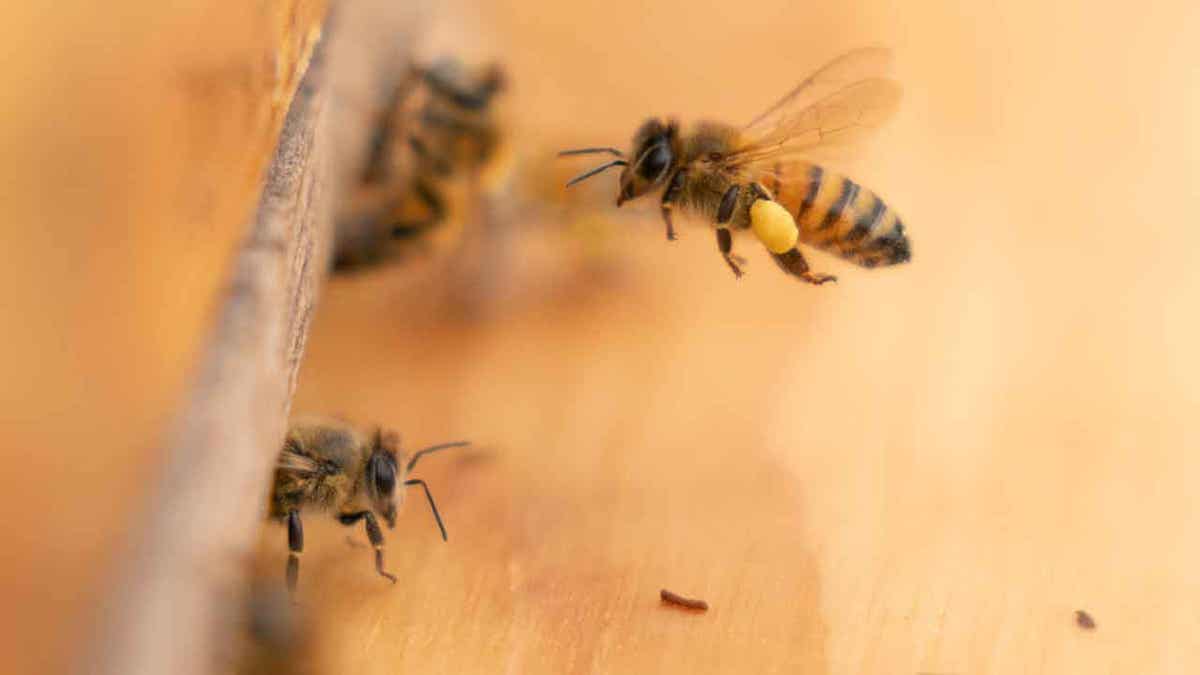This detailed, close-up color photograph captures several honeybees near a horizontally rectangular, polished wood log, which spans from the left to the center of the image. The background exhibits a gradient transition from an orange hue in the left center to a beige shade on the right. Notably, two bees are emerging from underneath the log on the darker brown left side, with one appearing blurry in the background. A prominent bee, sharply focused, is hovering near the center top, facing left, with its transparent wings in motion. This bee showcases striking features: black antennae, a large black eye, and a body adorned with alternating yellow and dark brown stripes. On its hind leg, there is a noticeable large yellow sac or cyst. Other elements in the image include a couple of small dark brown specks on the wood and various minor smudges, contributing to the natural, outdoor ambiance of the scene.